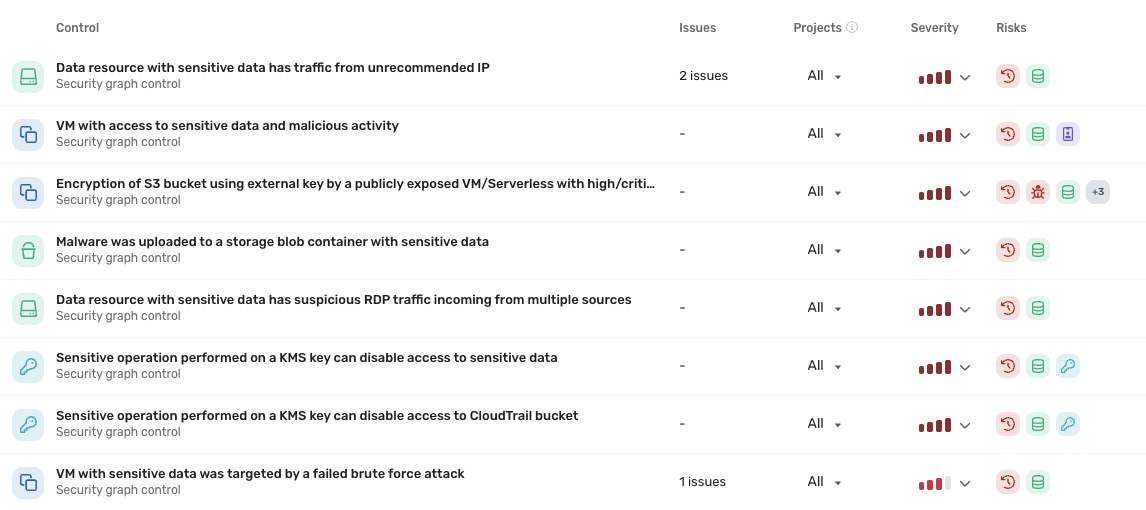In this detailed image, the background is white, featuring a structured table with five columns. The columns are labeled from left to right as: Control, Issues, Project, Severity, and Risk. Each row in the table details specific security concerns and issues. 

- At the top left, the label "Control" is prominent. 
- **Row 1** outlines a "Data resource to sensitive data has traffic from unrecommended IPs." There are two issues listed under "Issues", the project is marked as "All", and the severity is depicted by a red (maroon) signal icon, with four fully filled bars indicating high severity. The Risk column features both red and green icons.
- **Row 2** describes a "VM with access to sensitive data and malicious activity," showing no issues under "Issues", with the project labeled "All". The severity level is high with a depiction of three icons.
- **Row 3** details an "Encryption of S3 bucket using external key by a publicly exposed VM or serverless with high critical". There are no issues noted, the project is indicated as "All", and the severity is high, described as high risk.
- **Row 4** addresses "Malware uploaded to a storage blob container with sensitive data," with no issues under "Issues". The project is "All", with high severity and high risk denoted.
- **Row 5** involves a "Data resource with sensitive data and suspicious RTP traffic incoming from multiple sources". It shows zero issues, with the project as "All", and both severity and risk marked as high.
- **Row 6** specifies a "Sensitive operation performed on a KMS key can disable access to sensitive data," with zero issues, project "All", and high severity and risk.
- **Row 7** repeats the KMS key issue, but this time it mentions it can disable access to a CloudTrail bucket, with similar severity and risk indicators.
- **Row 8** mentions a "VM with sensitive data was targeted by a failed brute force attack," indicating one issue, with the project as "All", and severity showing three out of four bars.

Each entry under the Control column includes the note "Security Graph Control" beneath it. The image's overall theme revolves around various security threats and their associated severity and risk levels, meticulously documented in a clean, white-backgrounded table.